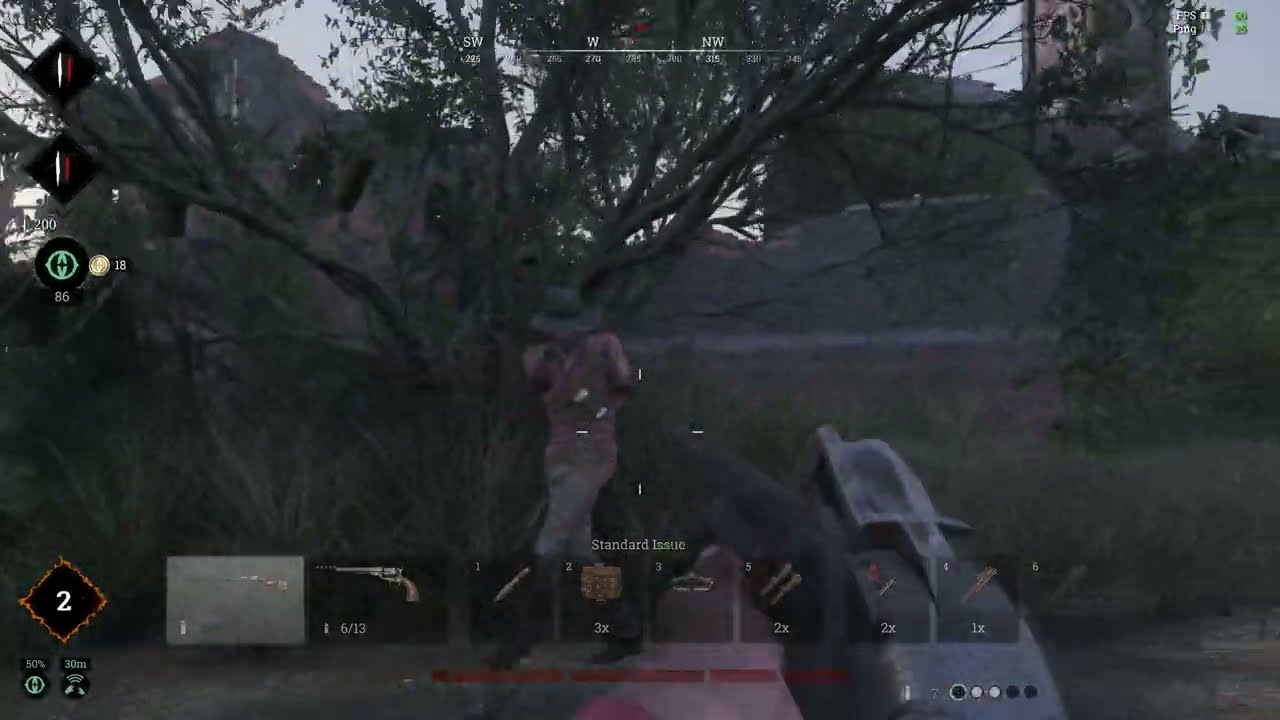This image is a screenshot from a first-person shooter video game with a Western theme, viewed from the player's perspective. The player is armed with an old shotgun or rifle, and crosshairs are pointed at an enemy figure ahead. The figure, wearing a hat and a light red shirt with off-white pants, is positioned near a tree amidst bushes, boulders, and rocks. They appear to be walking left, possibly holding weapons, with shell casings visible in mid-air. The landscape includes trees, bushes, and a distant rundown fortress or castle under a blue sky.

The user interface is detailed with various elements: a compass at the top center to show direction, and black diamond-shaped icons with tally marks and a circle labeled "B6" with a coin marked "18" on the right. The bottom left features a black diamond with an orange outline labeled "2." Along the bottom, the player's inventory is displayed, including an assault rifle, a long pistol, a knife, possibly a crowbar, a backpack, and other items, each indicating available ammunition or quantity.